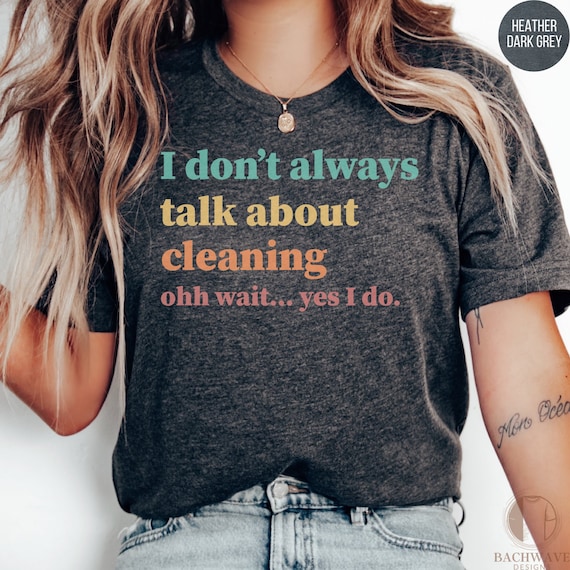The image is an advertisement for a t-shirt featuring a heather dark gray design worn by a woman with long blonde hair. Her head is cut off, showing only the area from her chin to just below her waistline. The woman appears to be very tan, has wavy hair, and is wearing a gold chain necklace with a pendant. The t-shirt displays a playful message in four lines of colorful text, progressing from teal to yellow, then orange, and finally pink, which reads: "I don't always talk about cleaning. Oh wait, yes I do." She is dressed in slightly faded blue jeans that are slightly tucked in at the sides, revealing the button in the center. The background is entirely white, casting the woman's shadow against it, and in the top right corner, a dark gray circle with the words "Heather Dark Gray" is visible. Additionally, there is a logo in the bottom right corner that reads "Back Wave Designs" accompanied by a drawing of a t-shirt. The woman also has visible tattoos on her left forearm, both below and above her elbow.